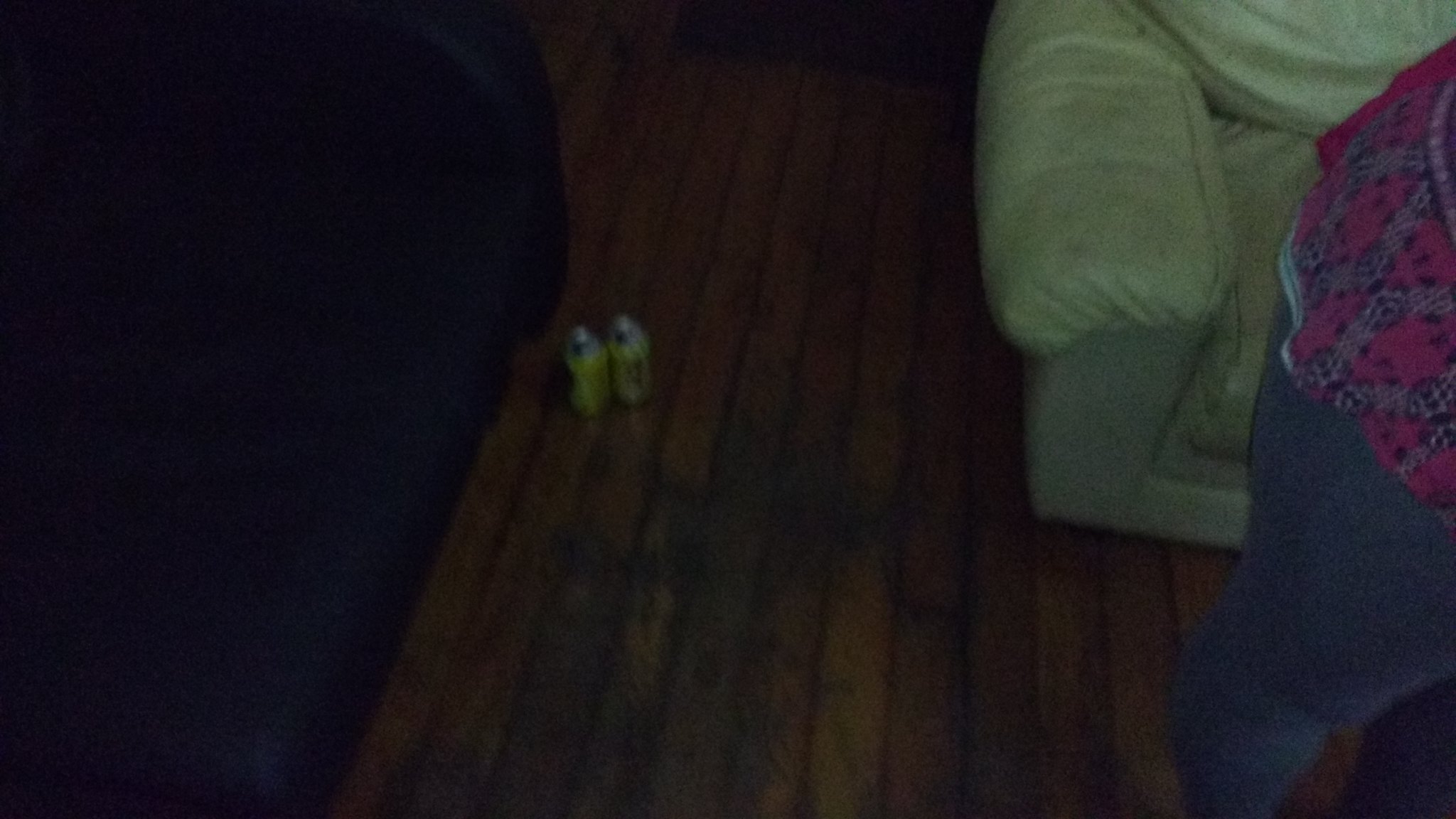In the image, a deceased creature lies on a brown wooden floor. The floor is strewn with two open green cans, their lids discarded nearby. On the left side of the frame, a piece of furniture, possibly a door or dresser, is partially visible. To the right, an old green chair with worn, folded fabric stands out; its material could be either deteriorated leather or heavily used fabric. A person is captured in the act of rising from this chair. They are dressed in blue jeans and a pink shirt featuring white and black stripes with white trim.